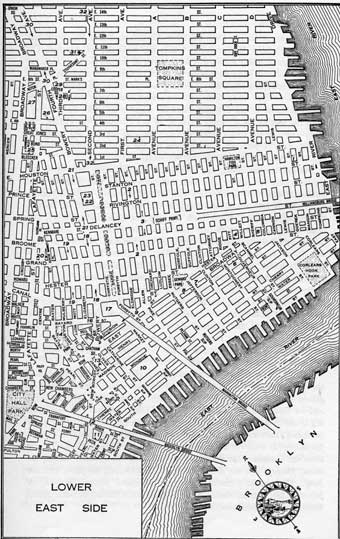This is a detailed, hand-drawn, black and white city map, likely from the early 1900s or the 1920s. The map prominently features the Lower East Side in the bottom left corner and Brooklyn in the bottom right. A compass, which is situated on land near the East River, points east and indicates different directions on the map. The East River, depicted in gray while the rest of the map is white, winds around the city, visible on both the lower and upper right sides of the map. The main section of the map is densely populated with numerous small rectangles arranged in lines, representing buildings. In the top middle, there is a distinct square area surrounded by these rectangles, potentially indicating a central plaza or significant landmark. Additionally, there appear to be people traversing the East River.